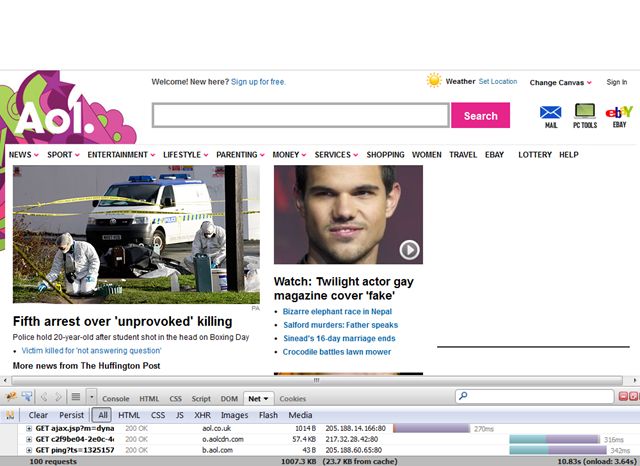The image displayed in the top left corner features a design in pink, purple, and green hues. Prominently, in white, it reads "AOL." The upper section of the image displays an enthusiastic "Welcome!" followed by the question "New here?" with an invitation to "Sign up for free." Below this text, there's a rectangular search box accompanied by a pink button on the side, which says "Search" in white text.

At the very top of the screen, a sun icon is present, indicating weather features. Additional options such as "Set location," "Change canvas," and "Sign in" are also available. To the right of the search box, several key functionalities are listed, including "Mail," "PC Tools," and "eBay."

Below these, there are several drop-down menus for categories including "News," "Sport," "Entertainment," "Lifestyle," "Parenting," "Money," and "Services." Further tabs labeled "Shopping," "Women," "Travel," "eBay," "Lottery," and "Help" are positioned beside the drop-down menus.

On the left-hand side of the image, a graphic resembling a crime scene photo is depicted. Beneath it, the headline states "Fifth arrest over unprovoked killing," followed by a subheadline: "Police hold 20-year-old after student shot in the head on Boxing Day." 

To the right of this, there's a picture of an actor with the caption "Twilight actor in fake gay magazine cover." Below this image are four bullet points in blue writing, which announce: 
- "Bizarre elephant race in Nepal"
- "Salford murders: Father speaks"
- "Sinead's 16-day marriage ends"
- "Crocodile battles lawnmower."

At the very bottom of the image, there are three lines that appear to contain some form of code. At the very bottom, it reads "100 requests."